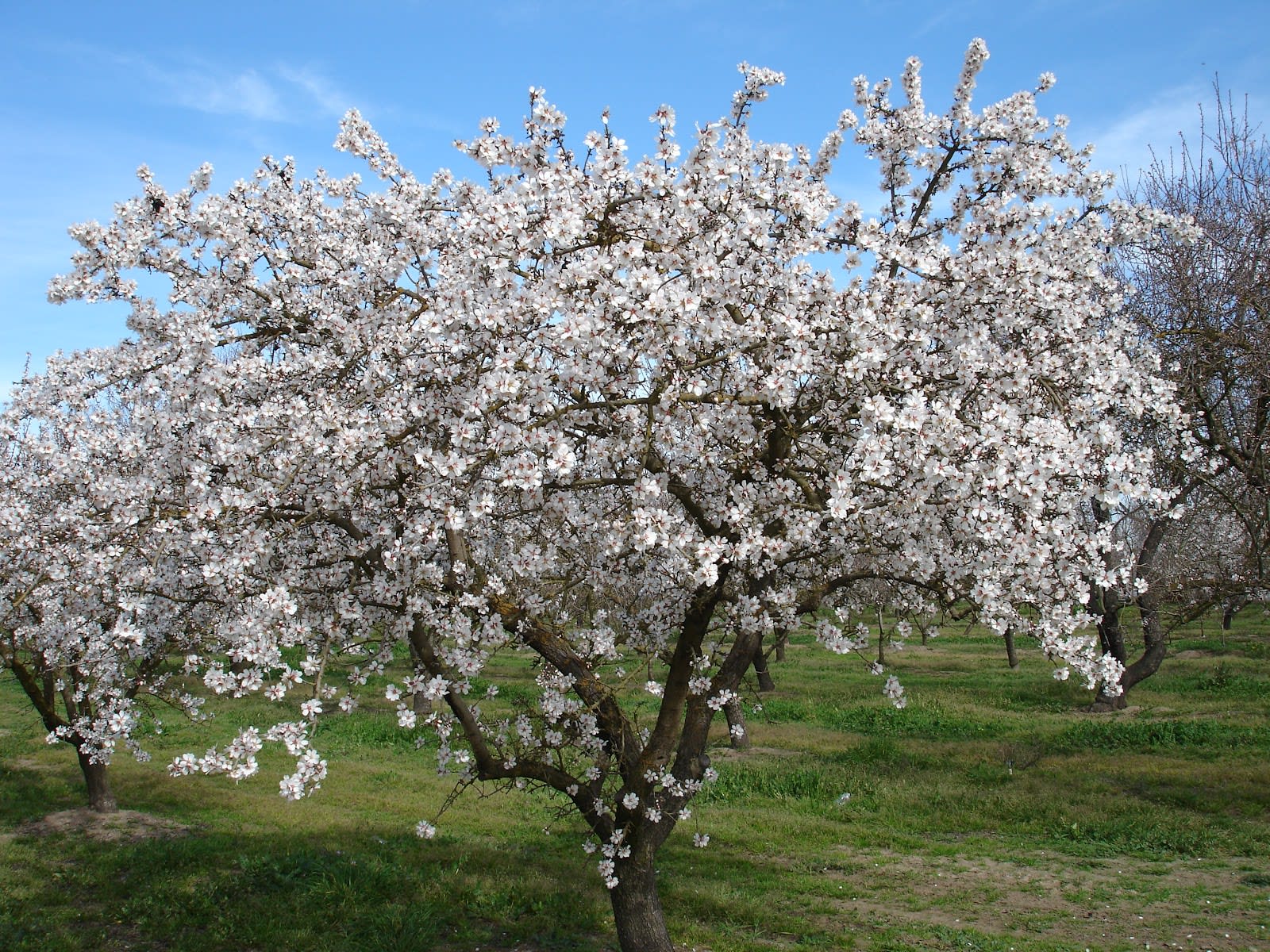This photograph captures a sunlit orchard, with a vibrant blue sky lightly dotted with wispy clouds as a backdrop. At the center, dominating the image, stands a medium-sized, wide-spreading cherry tree in full bloom. Its branches, extending outward, are densely covered with delicate white blossoms displaying a subtle blush at their centers, showcasing the peak of springtime beauty. Below, the ground is a mix of green grass interspersed with worn patches of dirt. In the background, hints of other tree trunks and branches suggest a methodical grid pattern, reinforcing the impression of an orderly orchard. Some distant branches lack blossoms, hinting at different tree varieties within the orchard. The scene is devoid of people and wildlife, emphasizing the serene and natural beauty of the blossoming cherry tree as the central focal point.